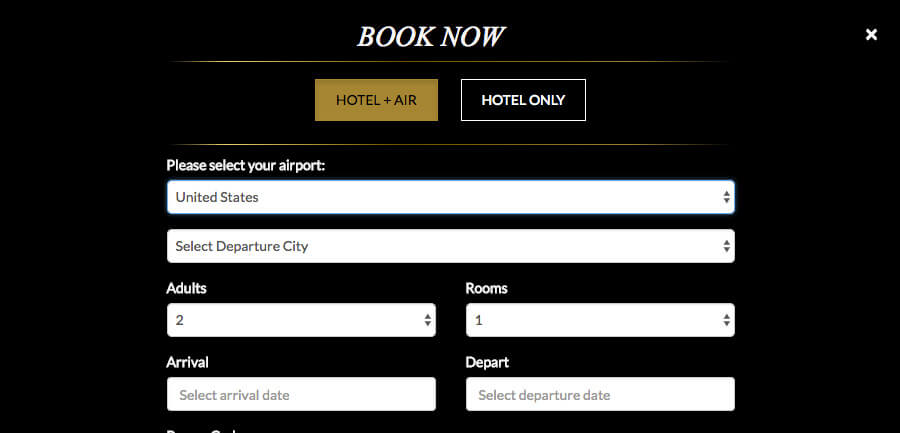The image features a black background with various interactive elements for booking a hotel and air travel. In the upper right corner, there's a bold, uppercase white "X" centered at the top, accompanied by the text "BOOK NOW". Below this, a yellowish-brown rectangular box contains the text "HOTEL + AIR" in all capitals. Adjacent to this is another informational box labeled "HOTEL ONLY".

On the left side, the text prompts users with "Please select your airport:" followed by a colon. Beneath this prompt, a long rectangle displays "UNITED STATES" with options to use the up or down arrow to select a different country. Further down, users can "Select Departure City" using another similar up and down arrow mechanism.

The form continues with fields for "Adults," prefilled with the number 2, and "Rooms," prefilled with the number 1. It also has a section for selecting travel dates: "Arrival" is indicated with an option to "Select Arrival Date". To the right of this is the word "Depart" and a white rectangle with light gray text stating "Select Departure Date", indicating that this field has not yet been clicked on.